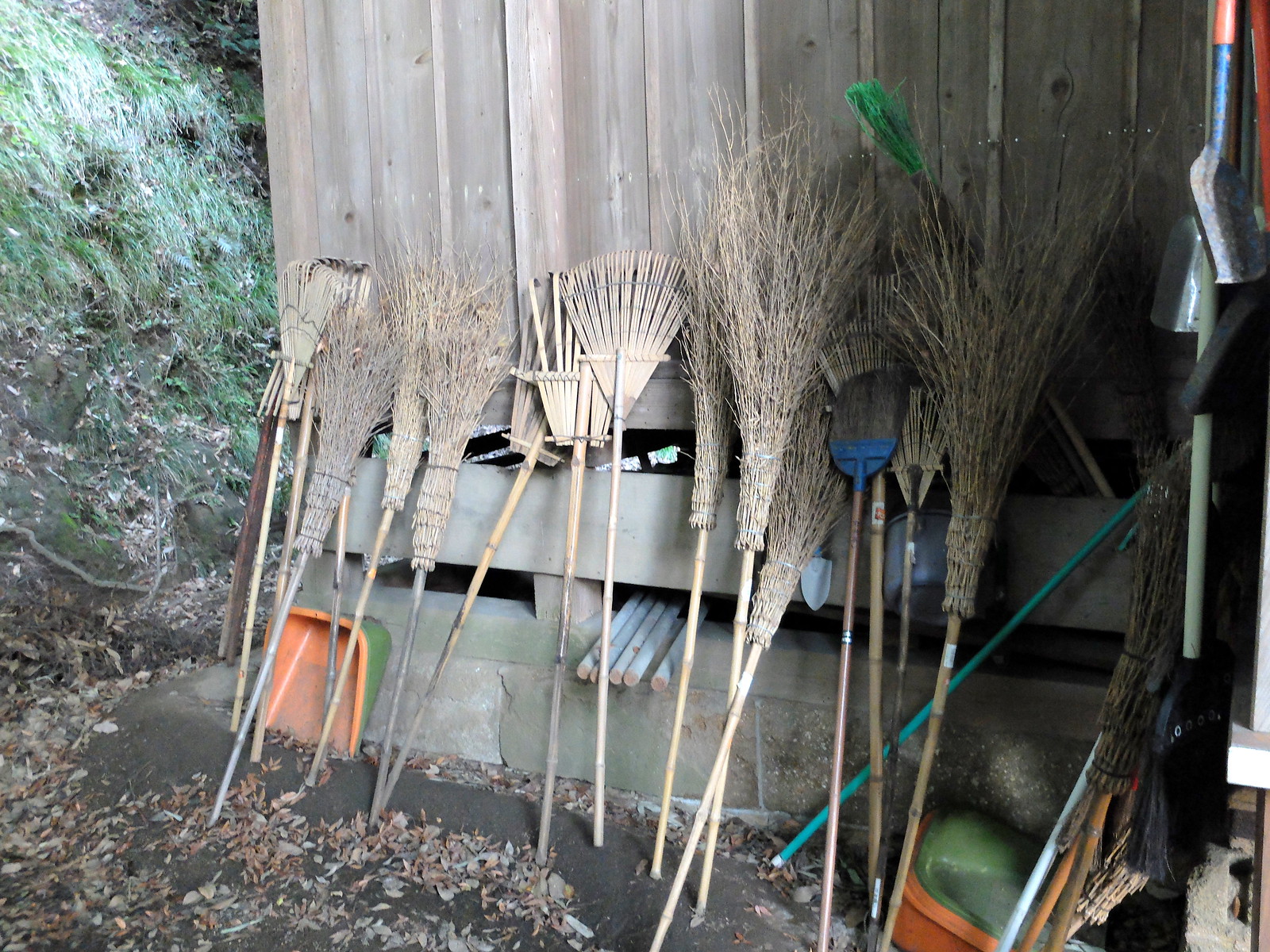This photograph depicts an assortment of yard tools leaned against the wooden side of a storage shed or barn. Prominently featured are various wooden rakes and brooms, some of which appear to be homemade. The brooms, resembling witches' brooms, are crafted from tied branches around a bamboo stick, while others are made from flat pieces of bamboo, mimicking the structure of a rake. The tools, primarily brown in color, suggest a natural, rustic aesthetic. In addition to these, there are orange plastic sweepers, likely used for gathering debris into buckets, which are visible on the ground amid scattered dry leaves. This eclectic collection of yard tools underscores a blend of functionality and handcrafted charm.